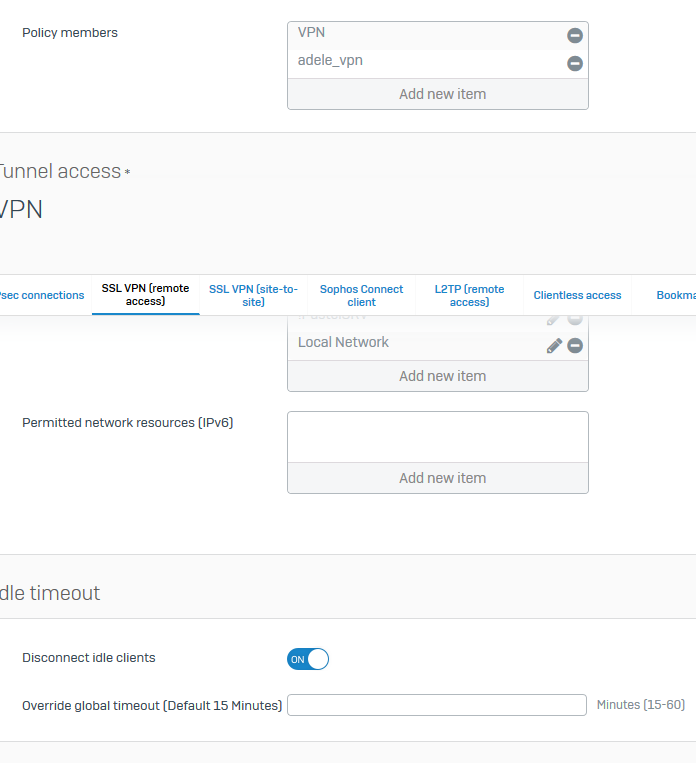Here is a cleaned-up and detailed caption for the image:

---

This image depicts a configuration page for setting up a Virtual Private Network (VPN) service. The page allows administrators to configure various VPN settings, including adding new items to the VPN setup. It features options such as "Tunnel Access," "SSL VPN Remote Access," "SSL VPN Site-to-Site," and "Client L2TP (Layer 2 Tunneling Protocol) Remote Access." Additionally, there's a "Clientless Access" option and sections to manage bookmarks.

Further down, the page presents settings for "Permitted Network Resources," enabling administrators to specify which network resources are allowed through the VPN. There are also controls for "Timeout Disconnect" settings, including parameters such as "Idle Timeout Disconnect," allowing adjustments to override the global default timeout (e.g., 15 minutes, 60 minutes). These settings determine how long a client can remain connected to the network without activity before being automatically disconnected.

Overall, this interface is designed to help network administrators set up and manage VPN connections, configure access permissions, and control connection durations to optimize network performance and security.

---